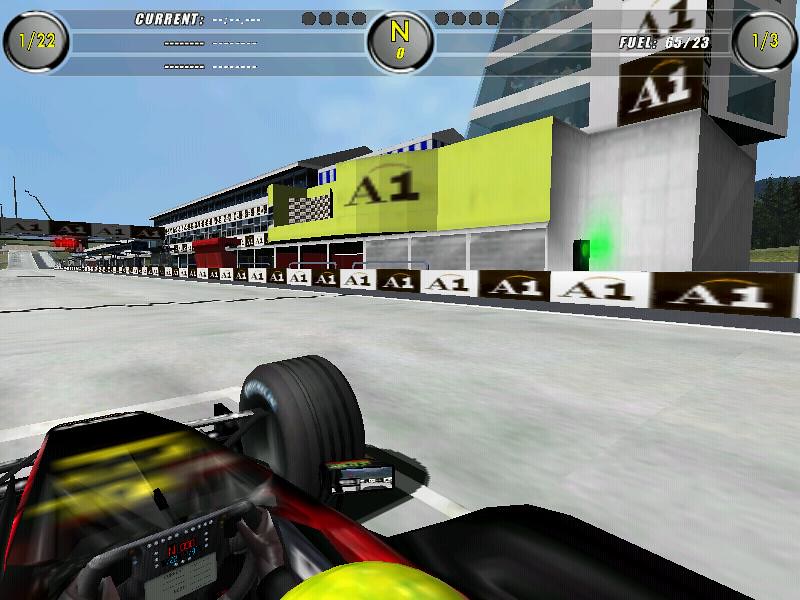This screenshot from a Formula One-style racing game showcases a car in pole position on a wide, gray racetrack. The camera angle is from above, looking down at the top of the driver's helmet, highlighting the front part of the red car and its steering wheel. The right front tire is visible, sticking out prominently due to the lack of a covering. The track is framed by a concrete building on the right, featuring a door with a green light and a large yellow section emblazoned with a black "A1." Alongside the track is a wall of alternating black and white rectangles also marked with "A1." The race has yet to start, as indicated by the "1/22" position display and other on-screen info, including symbols for fuel and lap count, showing this is the first lap in a three-lap race. The bright blue sky adds to the game's vibrant atmosphere.